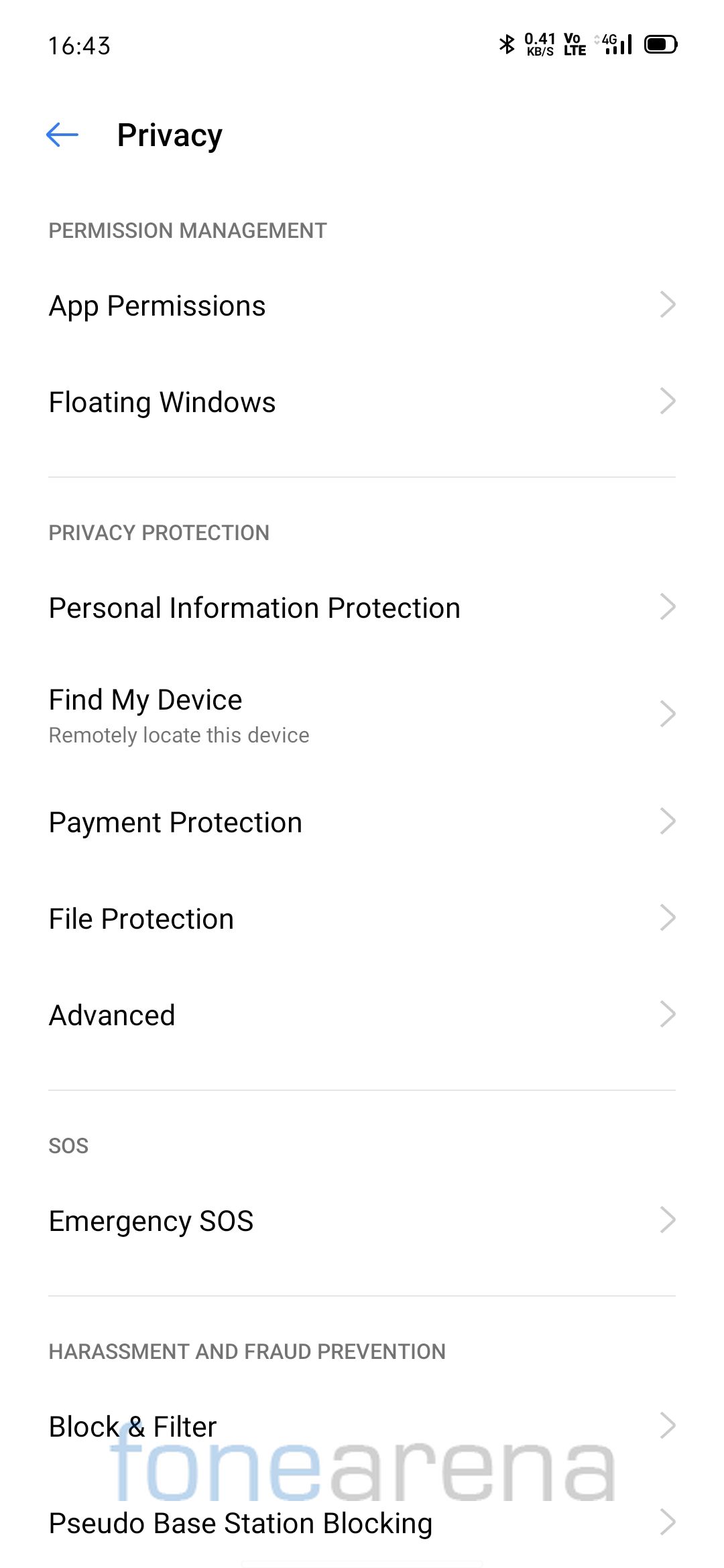The image displays a user interface screen with the following details, organized from top to bottom:

1. **Time:** The screen shows the time as 16:45.
2. **Battery Status:** The battery icon indicates that approximately three-quarters of the battery is remaining.
3. **Navigation and Section Titles:**
   - A blue arrow pointing to the left.
   - Bold black text reading "Privacy".
   - Smaller gray capital letters stating "PERMISSION MANAGEMENT".
   - Larger black text reading "App Permissions".
   - Text "Floating Windows" followed by a light gray line spanning left to right.
   - Gray capital letters stating "PRIVACY PROTECTION".
   - Bold black text reading "Personal Information Protection".
   - Text "Find My Device".
   - Gray text explaining "Remotely locate this device".
   - Bold black text reading "Payment Protection".
   - Text "File Protection".
   - Text "Advanced".
   - Small gray capital letters stating "SOS".
   - Bold black text reading "Emergency SOS".
   - Gray small capital letters stating "HARASSMENT AND FRAUD PREVENTION".